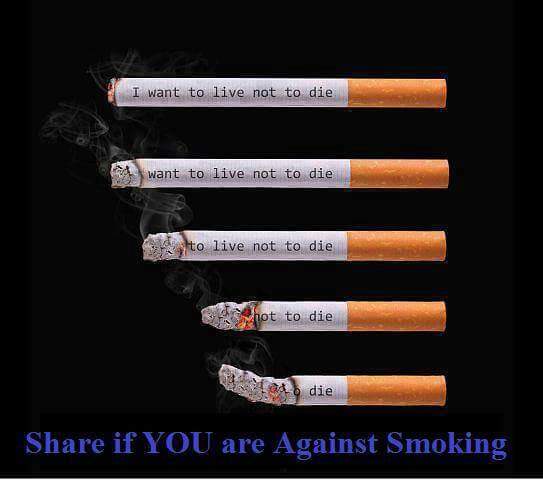This anti-smoking campaign poster features a striking visual on a black background. It displays five cigarettes, each at a progressively advanced stage of being burnt from left to right. The first cigarette is barely lit and is accompanied by the phrase "I want to live, not to die." The next cigarette, burned slightly more, has the words "Want to live, not to die." As the cigarettes burn down further, the third says "To live, not to die," the fourth reads "Not to die," and the final, most burnt, simply states "Die." This stark progression underscores the deadly consequences of smoking. At the bottom of the poster, in blue lettering, is the call to action: "SHARE IF YOU ARE AGAINST SMOKING," with "YOU" emphasized in all capital letters, urging viewers to spread the anti-smoking message.